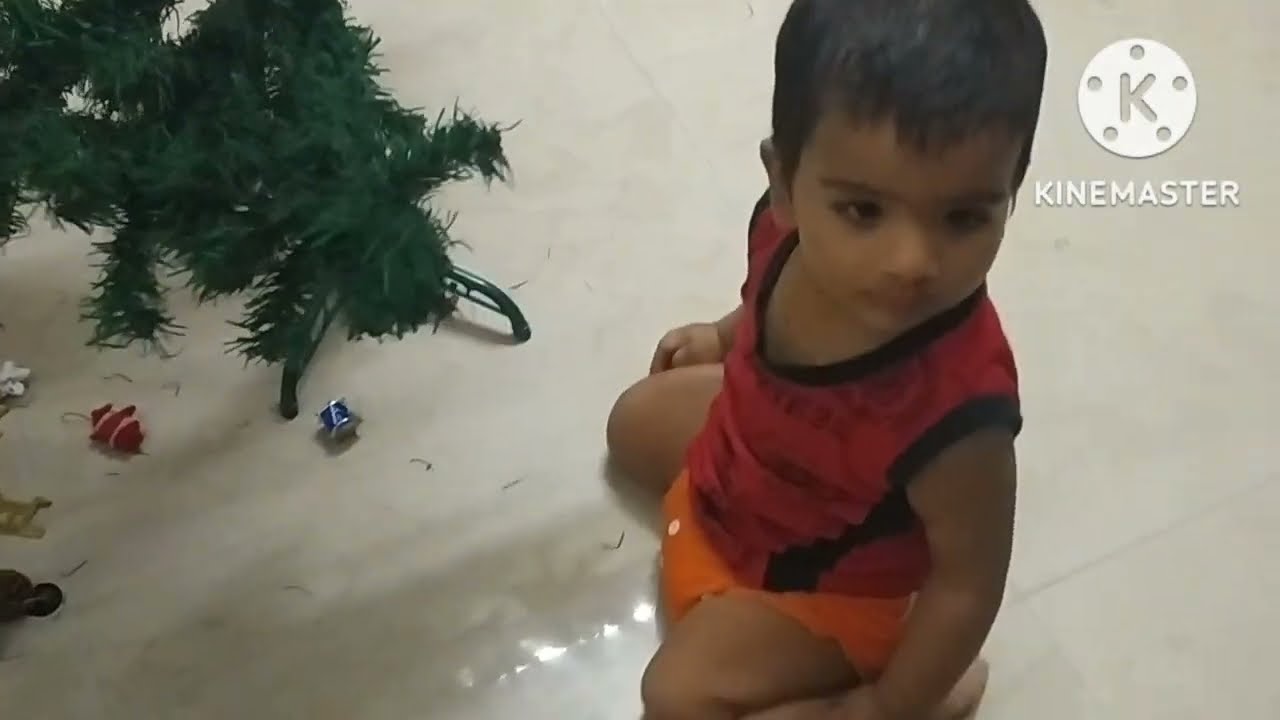In the image, there is a young boy with dark skin and short black hair, captured looking slightly away from the camera. He is wearing a sleeveless red tank top with black trim around the neck and armholes, paired with orange shorts. The boy is kneeling on a shiny, white floor, in front of a Christmas tree. The tree is a bit bent, and several ornaments, including white, red, blue, and black ones, are scattered on the floor around him. The upper right corner of the image features the text "KineMaster" with a white circle surrounded by five dots and a 'K' in the center. The scene appears to be indoors, likely in a home setting, and evokes a Christmas theme.